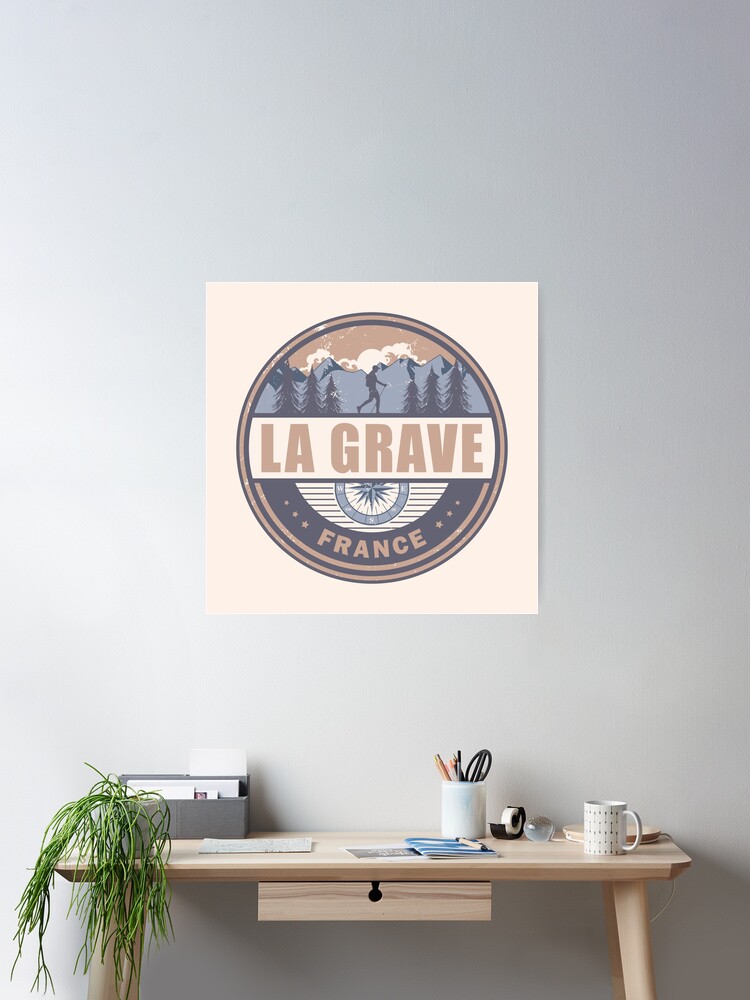The image depicts a minimalist and aesthetically pleasing desk setup against a pristine white wall, bathed in light from the left. Central to the scene is a prominent poster that reads "La Grave, France," featuring an illustration of mountains and trees with a man in the center holding a cane or ski pole, suggesting a hiking area. Above the text "France" is a design element composed of blue lines forming a circle, possibly a compass, and light red rings. The desk itself is a simple wooden piece, likely from a store like Ikea, featuring a small drawer. On the desk, there is a small compartment for organizing paperwork, a wilting potted plant on the left, a Pixar-style lamp, a coffee mug, a tape dispenser, a little pencil bowl, and some paper with writing on it. This organized yet inviting workspace is both functional and visually appealing.